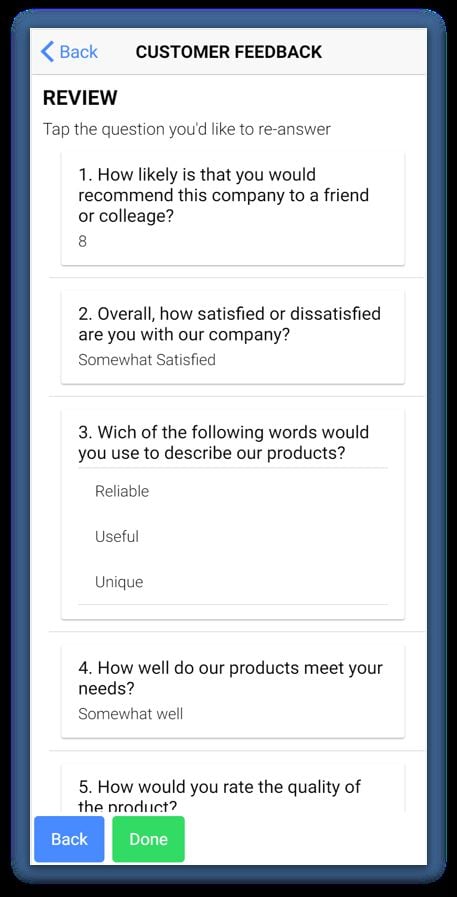The image features a stark white background with a navigation element at the top displaying a "Back" arrow, represented by a less-than symbol ("<"). The primary content of the image appears to be centered around customer feedback and review prompts. 

The first section poses the question: "How likely are you to recommend this company to a friend or colleague?" with a respondent rating it as an "8" out of a possible higher value. The second question addresses overall satisfaction with the company, to which the respondent marks as "Somewhat satisfied".

The third question seeks descriptors for the company's products, offering options like "Reliable," "Useful," and "Unique." Following this, the fourth query asks how well the company's products meet their needs, with the respondent indicating "Somewhat well."

For the fifth and final question, the quality of the product is to be rated, although no specific response is provided in the text.

At the bottom of the image, there are two prominent buttons for navigation and submission purposes. A blue rectangle labeled "Back" in white text allows users to navigate to the previous section. In contrast, a green rectangle labeled "Done," also in white text, indicates the completion of the feedback submission.

Overall, the image clearly depicts a structured customer feedback form with intuitive navigation and response options, set against a clean and minimalist design.